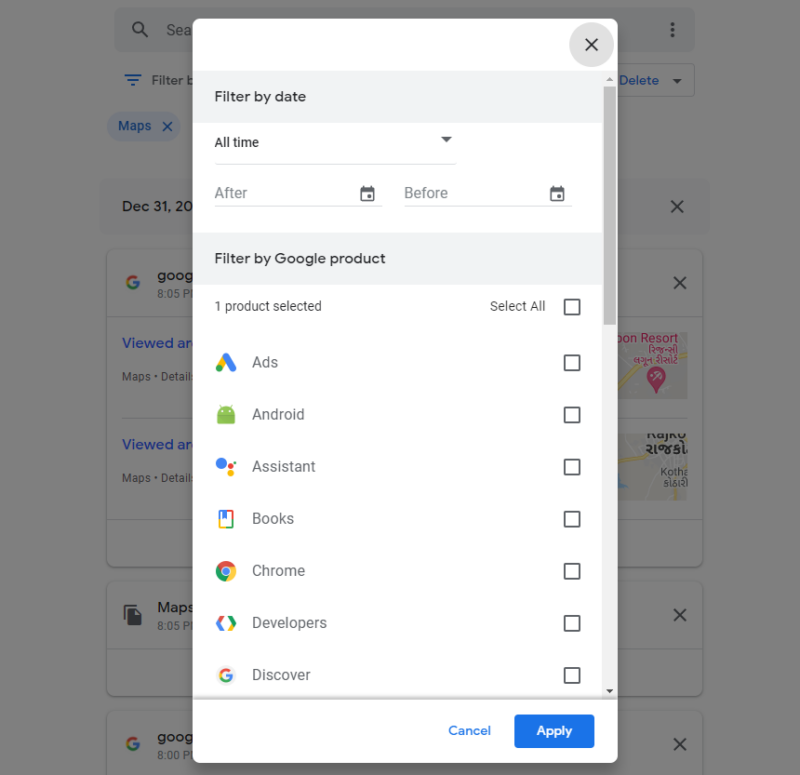A screenshot shows an interface from a website, where an overlaid menu obscures the underlying page, which appears to contain some partially visible Google-related content. The background is grayed out to highlight the white, portrait-oriented overlay box in the foreground. This overlay contains several interactive elements.

At the top right corner of the overlay, there's an "X" button to close the menu. Below it, a gray banner displays the text "Filter by date." Users can filter results using various date options such as a dropdown menu labeled "All time" and fields to select "after" and "before" dates, each accompanied by a calendar button to facilitate date selection.

Another gray banner below reads "Filter by Google product." Underneath, it states "1 product selected," though seven different selectable options are listed: Ads, Android, Assistant, Books, Chrome, Developers, and Discover. Each option has an associated icon on the left and an unchecked white checkbox on the right.

Toward the bottom of the overlay, a thin gray banner separates the main fields from two buttons aligned to the right: a blue "Cancel" button and a blue "Apply" button. This layout suggests a filtering process for customizing search results or settings before returning to the main page.